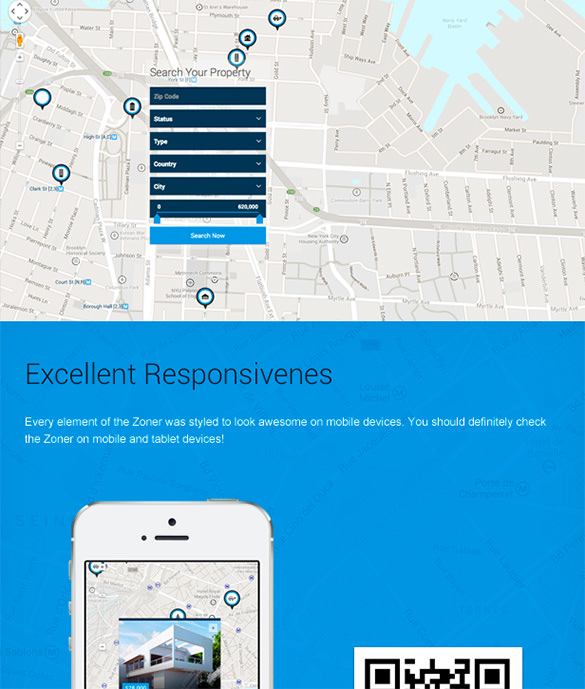This image is a screenshot featuring a split layout with a map interface and an advertisement. 

**Top Half:**
Dominating the top section, the map includes various markers, each adorned with distinctive icons. Near the center of this map, there's a horizontal cutoff where the advertising image starts. Above this cutoff, the map includes a control panel with a series of buttons that allow the user to filter search results. These buttons include options for "Zip Code," "Type," "Country," and "City," which are all drop-down menus for refining the search criteria. At the top of this panel, a prompt labeled "Search Your Property" guides the user to the function available. Beneath these drop-down menus, a prominent blue button labeled "Search Now" invites the user to initiate the search.

**Bottom Half:**
Occupying the lower part of the screen, the advertisement champions "Excellent Responsiveness." This segment features an image of a smartphone displaying a QR code, suggesting a modern, interactive feature that users can scan for additional information or resources.

This detailed layout effectively merges the functional aspects of a property search tool with an engaging, mobile-friendly promotional message.